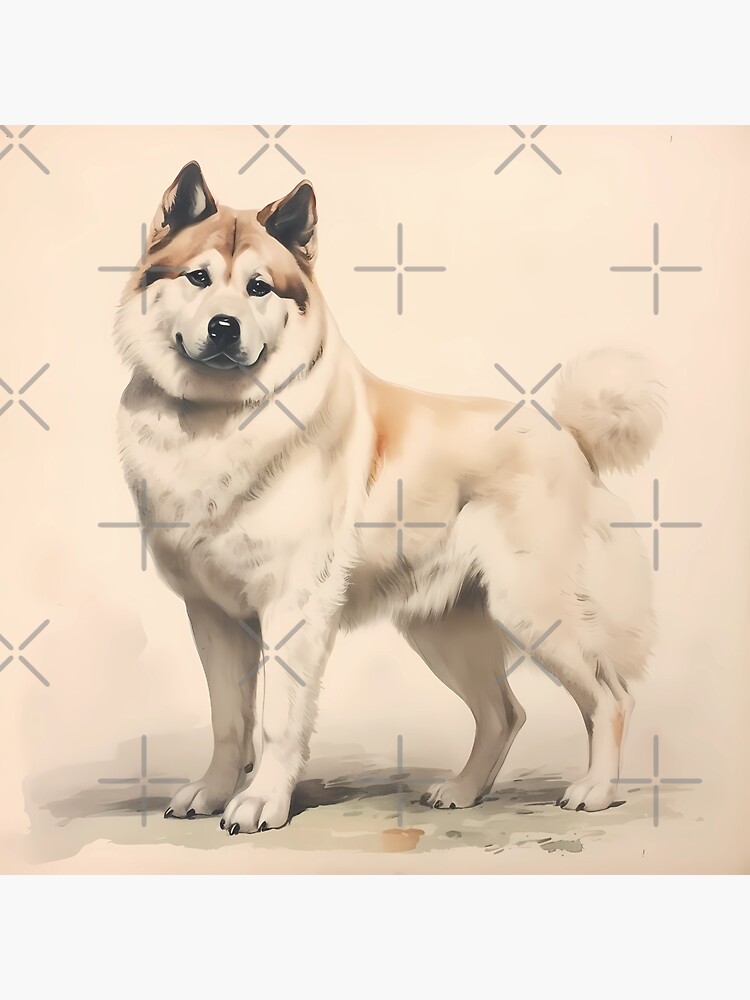This is a detailed watercolor illustration of a husky or malamute dog, presented in a square format. The dog stands in profile with its body facing sideways, but its head turned toward the viewer, giving an impression of engagement. It has pointed ears and a pointed muzzle with a shiny black nose and rounded dark eyes that contribute to an almost smiling expression. The coat is predominantly white with patches of beige, extending from the top of its head and around the sides of its face. Beige fur continues along its back and appears on the rib cage area, while the chest, legs, and puffy tail are primarily white. A slight rust or light tan shade can be seen going down its back and possibly along the hind legs. The background features a peach-colored base adorned with a repetitive pattern of faint gray crosses or X's, giving it a textured appearance. Shadows in tones of purple, green, and beige beneath the dog suggest the illustration's depth. The overall image has an artistic, possibly hand-painted feel, capturing the charm and sturdiness of the dog with its thick fur and softly blending colors.